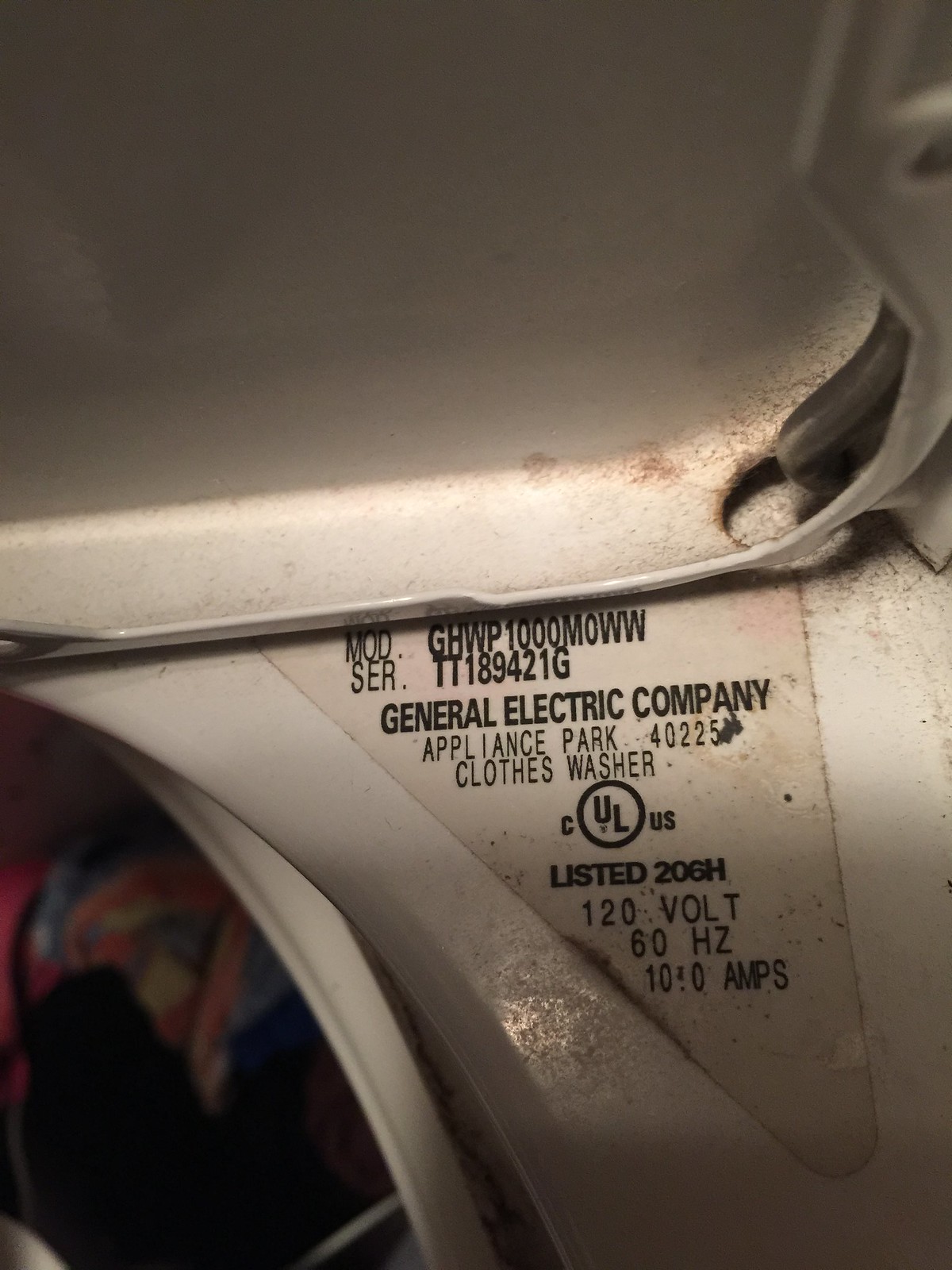The image depicts a close-up view of a washing machine, particularly focusing on a sticker with important information. The upper background features a gradient from khaki brown to a pinkish hue. The visible portions of the appliance are white metal, suggesting the machine's side door or frame. There is a round opening, presumably where clothes can be seen partially thrown inside. The detailed sticker on the machine displays the following: "MOD: GHWP1000MOWW" for the model number, "SER: TT189421G" for the serial number, "General Electric Company, Appliance Park, 40225," identifying the manufacturer and location. It further lists "Clothes Washer," confirming the appliance type, followed by specifics such as "Listed 206H," "120V," "60Hz," and "10.0A," which denote electrical specifications. The text on the sticker is black, and its worn appearance suggests it has been in place for a significant duration.